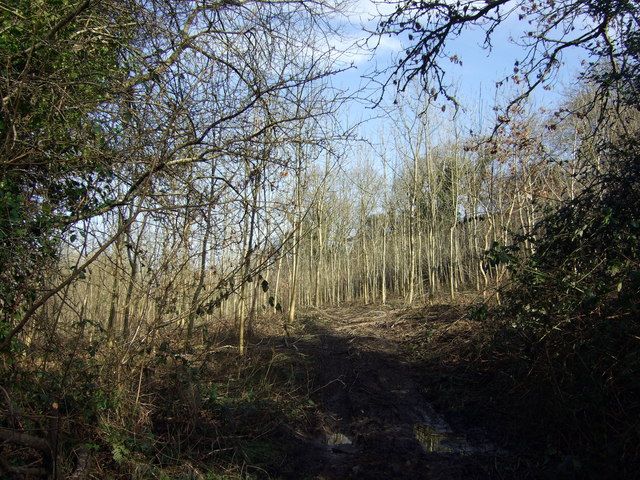This image portrays a serene forest landscape, primarily focusing on the natural environment rather than specific objects. The foreground features a ground covered with dirt, sticks, fallen leaves, and underbrush. Scattered bushes and branches create a dense, untidy undergrowth. The scene is characterized by numerous thin trees; many are leafless, though some have sparse foliage. A path winds into the depth of the forest, surrounded by clusters of trees on both sides. The lighting appears to transition from dim in the immediate foreground to brighter as one looks further into the image. Dominating the upper part of the image is a clear blue sky with wispy white clouds, adding a tranquil backdrop to the otherwise muted colors of the forest scene that include shades of blue, green, brown, gray, and black. This picturesque view captures the essence of a forested area, illustrating both the rich complexity of the underbrush and the open sky above.